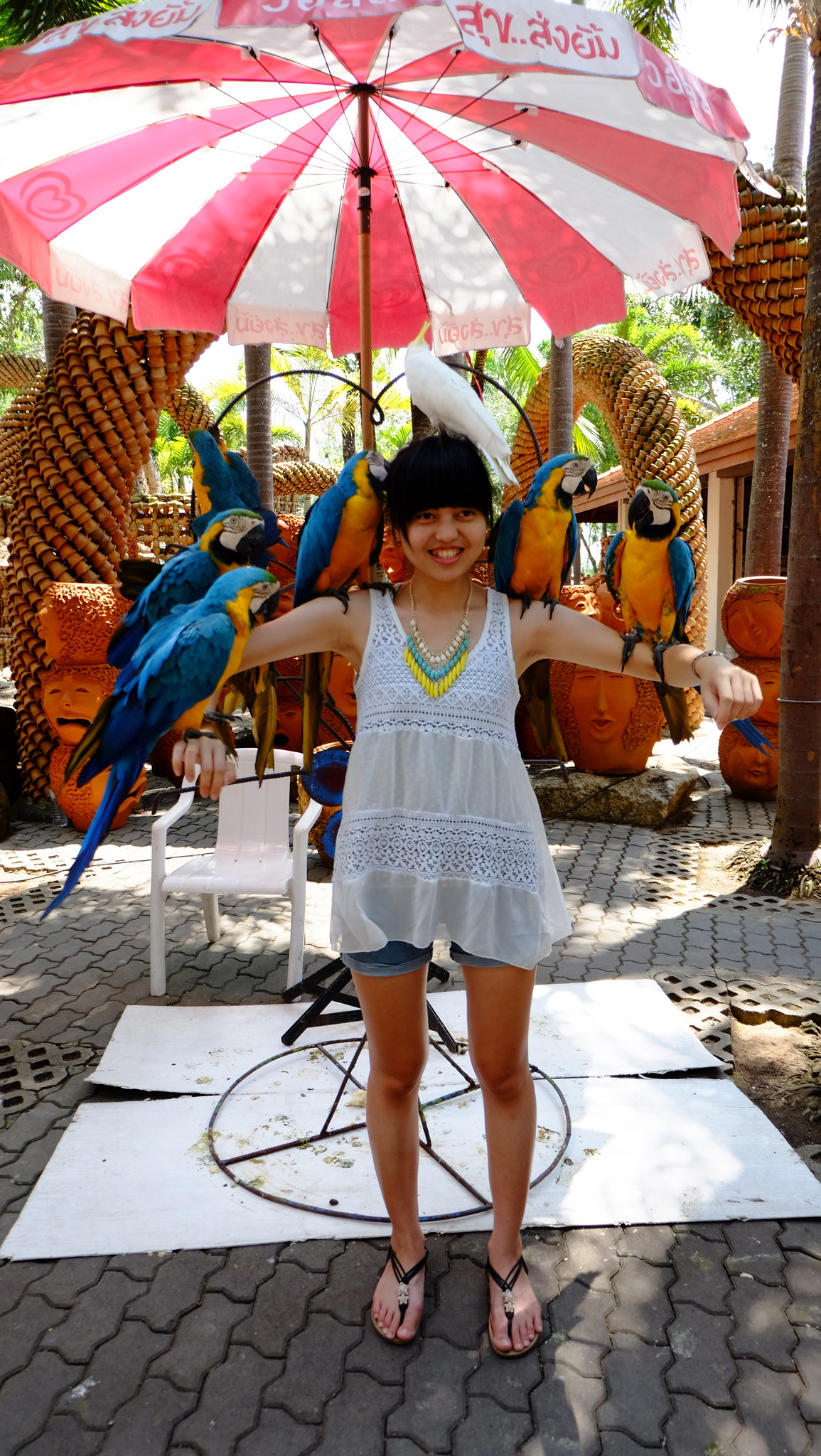In this vibrant daytime outdoor photograph, a young girl, possibly of Filipino or East Asian descent, stands smiling beneath a red and white umbrella. Her dark black hair is cut in a bowl style with bangs, and she wears a loose white blouse over blue denim shorts along with black sandals. Adorning her neck is a white, blue, and yellow necklace. The girl holds her arms outstretched, proudly displaying a collection of colorful parrots and parakeets perched along both arms. These birds feature blue heads, green accents around their faces and eyes, yellow-orange chests, and some show red under their wings.

She is positioned on a cobblestone or tiled pathway, surrounded by a backdrop that includes palm trees, various statues with facial features, and pine cone-shaped decorations. This lively scene, possibly set in a tropical location such as Hawaii, lacks any text or print, allowing the vivid colors and details of the setting to captivate the viewer's attention.